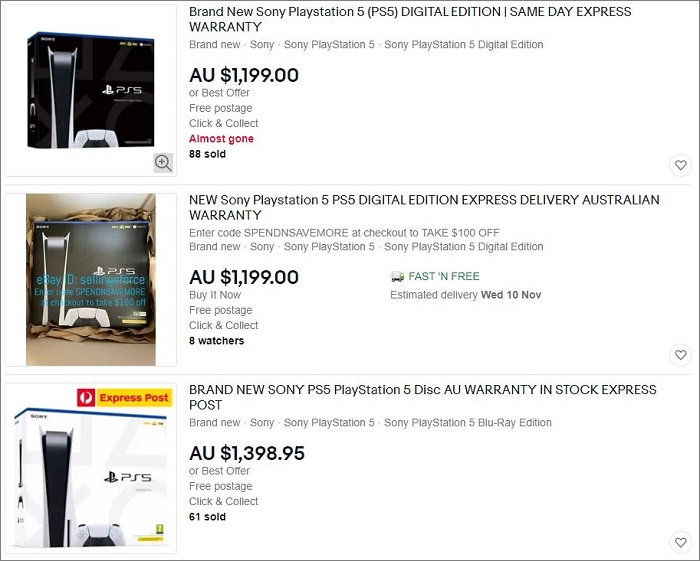This image is a detailed screenshot of a shopping website, featuring three distinct product listings vertically aligned. 

1. The first section displays a PlayStation 5 in a black box. The product is labeled as "Brand New Sony PlayStation 5 Digital Edition" with additional details indicating "Same Day Express Warranty." It is priced at $1,199 AUD or best offer, with free postage and a "Click and Collect" option. The listing is marked in red as "Almost Gone" with 88 units sold.

2. Below it, the second product listing also features a PlayStation 5, described as "New Sony PlayStation 5, PS5 Digital Edition" offering "Express Delivery" and "Australian Warranty." It includes a special promotion: entering the code "SPENDANDSAVE" at checkout grants a $100 discount. This item is priced similarly at $1,199 AUD, with "Fast and Free Shipping" and an estimated delivery date of Wednesday, 10 November. The listing indicates that eight people are watching this item.

3. The bottom section presents another PlayStation 5, but this time in a white box. Highlighted in yellow, the listing mentions "Express Post." The product title reads "Brand New Sony PS5, PlayStation 5 Disc" with "AU Warranty and Stock, Express Post." The item is listed at a higher price of $1,398.95 AUD and notes that 61 units have been sold.

Each listing provides specific details about warranties, shipping options, pricing, and sales performance, catering to different buying preferences and urgencies.